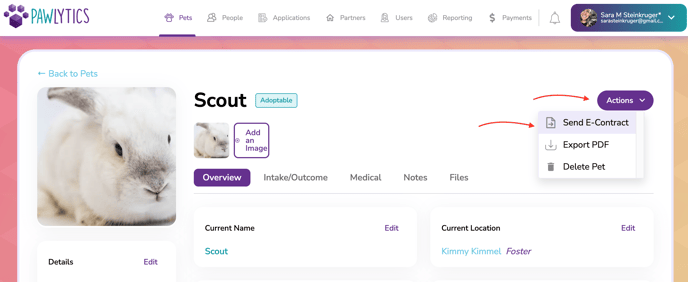This screen capture showcases a computer monitor displaying a predominantly white page from the Paw Lytics website. In the upper left corner, there's a logo featuring a purple paw print with four toes next to the site name written as "Paw" in blue and "Lytics" in purple. Centered at the top is a navigation bar with various tabs: a cat icon labeled "Pets," a "People" tab featuring two gray figures, an "Applications" tab with a square icon, a "Partners" tab with a house icon, a "Users" tab that is illegible in gray, a "Reporting" tab with a gray circle, a "Payments" tab marked by a gray dollar sign, and a gray notification bell.

In the top right corner, there's a rectangular user information bar displaying an image of a person and the name "Sarah M. Stein Kruger." Below this bar is a pink-framed window with a central white background. The top left corner of this window features a "Back to Pets" link in blue. Beneath it, a large square picture of a white rabbit face is prominently displayed. To the right of this image, the name "Scout" appears in black lettering next to a blue "Adoptable" bar. A thumbnail of the same rabbit image is followed by an "Add an Image" link.

Additionally, several clickable categories are listed: Overview, Intake, Outcome, Medical Notes, Files. The rabbit's current name is "Scout," and its current location is "Kimmy Kimmel Foster." On the right-hand side, there is a prominent purple "Action" button with an adjacent orange arrow. Another section beneath this contains a "Send eContract," "Export PDF," "Delete Pet" options, each highlighted by another orange arrow.